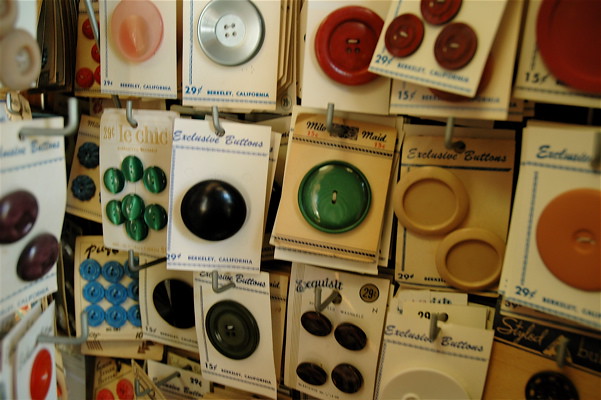The image captures an intricate display inside a store, showcasing a vast assortment of buttons for sale, mounted on cardboard backings. The assortment includes both large and small buttons in a wide spectrum of colors—silver, white, vibrant red, metallic green, light blue, orange, various shades of brown, pink, and more. These buttons are affixed on worn-out tan or light-colored cardboard cards, some holding just one large button while others feature several smaller ones. Each card is meticulously hung on metal hooks attached to wall paneling, with some displaying a price of 29 cents, and labeled "Berkeley, California." The buttons come in diverse shapes and styles, with some featuring four, two, or no holes at all. The display extends across three visible rows, with additional rows peeking from the lower left corner, indicative of an extensive and detailed collection perfect for any sewing and craft enthusiast.